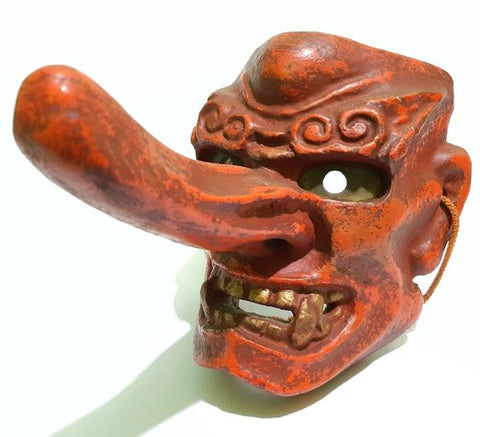This image features a striking and detailed red mask that appears to be crafted from stone and is reminiscent of an ancient artifact or festival mask. The mask has a distinctive, extremely elongated nose, almost twice the size of the mask itself, which protrudes prominently from the face. The red paint adorning the mask has a brushed texture and appears worn, giving it an aged look. The mask features greenish-brown eye sockets with white centers and a set of yellowish teeth that resemble fangs, adding to its fierce appearance. Additionally, there is a clear reddish strap visible on the back, indicating it was designed to be worn. The forehead is notably large and has a prominent lump, embellished with swirling designs around the area. A string extends from the mask’s ear, contributing to the intricate details. The background of the image is white with a hint of shadow at the bottom that has a slight greenish tint, giving depth to the photograph. Despite its serene background, the mask exudes a powerful presence, capturing the essence of a large, intimidating, and angry figure.